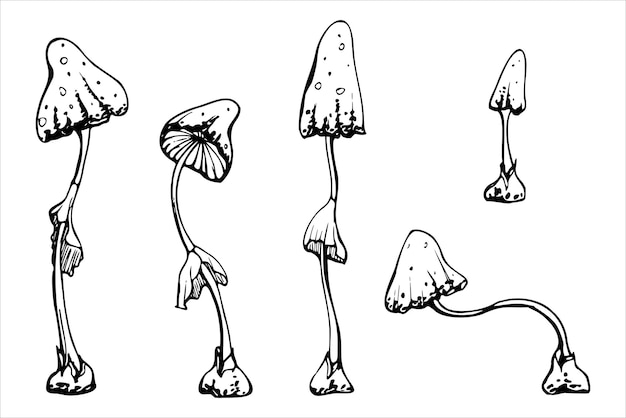This black and white drawing depicts five distinct mushrooms with tall, slender stems and caps reminiscent of shiitake mushrooms. Each mushroom varies in height, shape, and orientation, with one notably forming an S-shape as it leans over. The mushrooms, which look almost ghost-like with hooded caps adorned with spots, have stems that surprisingly feature leaves. Three of the mushrooms are clustered together on the left, another one stands slightly apart in the back, and the dramatically leaning mushroom occupies the foreground. The scene is set against a plain white background, emphasizing the unique forms and details of the mushrooms.